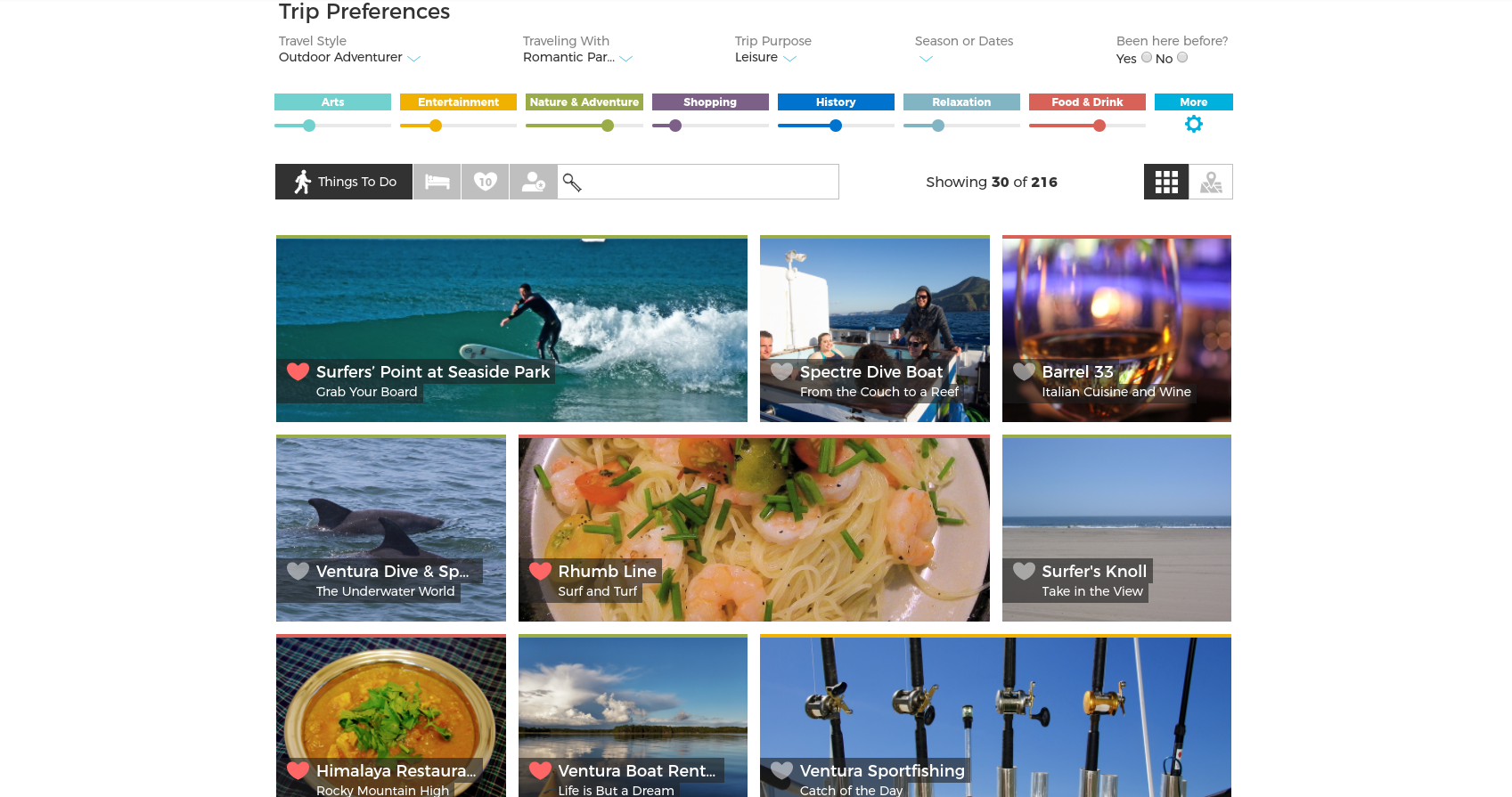**Detailed Caption:**

This image illustrates a travel planning website tailored for outdoor adventurers. The website offers customizable trip preferences, allowing travelers to select their travel style, which includes options such as traveling with a romantic partner, for leisure, or as an outdoor adventurer. Additional preferences like season or dates and whether the user has visited the destination before are also available.

Categories for various activities are displayed with colorful icons at the top, including Arts, Entertainment, Nature, Adventure, Shopping, History, Relaxation, Food and Drink, and more. A prominent search bar with a magnifying glass icon aids in finding specific activities. The user is currently viewing 30 of 216 suggestions for things to do.

Highlighted activities include:
- **Surf's Point at Seaside Park:** Featuring a man surfing ocean waves, which the user has liked, indicated by a red heart.
- **Spectra Dive Boat:** An adventure from the couch to the reef.
- **Barrel 33:** An Italian cuisine and wine venue, showcased by an image of a wine glass in the background.
- **Ventura Dive:** Promising an underwater exploration with dolphins.
- **Room Line Surf and Turf:** An eatery serving a pasta and shrimp dish, which the user has also hearted.
- **Surfers Know and Himalayan Restaurant:** Highlighted with a hearty red heart, the image shows an orange soup garnished on top — an allusion to its Rocky Mountain highs.
- **Ventura Boat Rentals:** Loved by the user, this activity is depicted with blue skies and water.
- **Ventura Sports Fishing:** Titled "Catch of the Day," the activity is illustrated with fishing reels poised upright in the daytime.

Each listed activity is marked with a small square image and the user’s preferences, as indicated by red hearts on their favorite options.